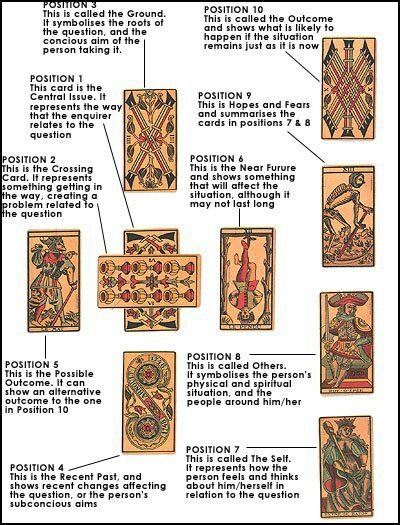This image is an instructional poster featuring a series of card-like rectangles that each depict different scenes. The layout is organized neatly against a white background, outlined with a black border, providing a clean and clear presentation.

Each rectangular card has an old-fashioned tan background and a unique scene depicted on it, adorned with colors predominantly in shades of red and blue, with minimal use of other colors. The scenes are accompanied by textual descriptions, which are meticulously placed to convey detailed information about each position.

The information for each card is formatted consistently: the word "POSITION" is written in all capital letters, followed by a number (e.g., POSITION 1, POSITION 2, up to what seems to be POSITION 10). Beneath each "POSITION" title, there is a paragraph written in sentence case that elaborates on the scene depicted in the corresponding card. 

A straight black line connects each paragraph to its respective card, ensuring clear association between the text and the visual representation. This systematic layout allows viewers to easily follow along and understand the depicted instructions or information being conveyed.